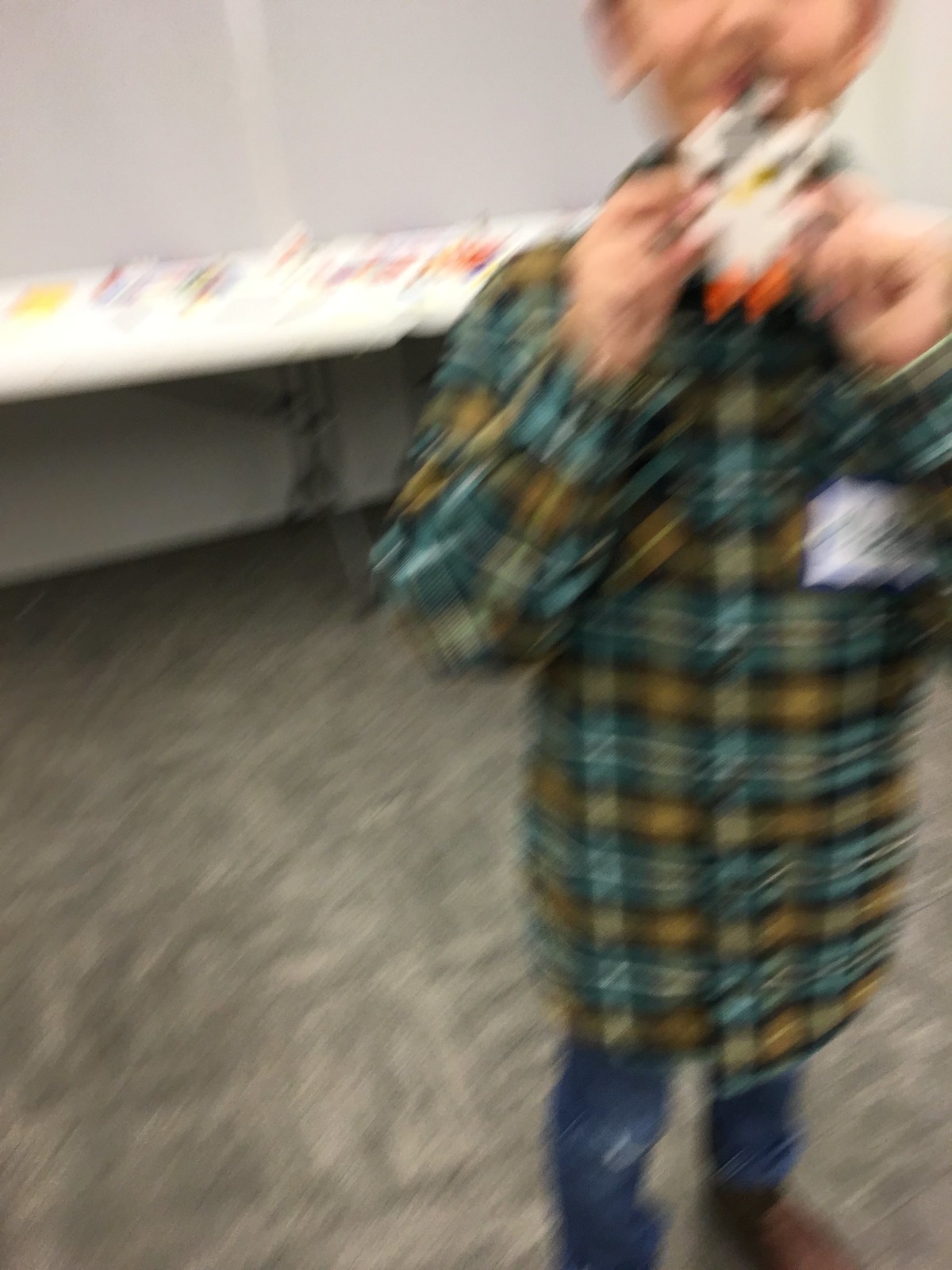In this blurry image, a young boy is partially captured, standing in what appears to be an elementary school classroom. The boy, who has light skin, is dressed in a plaid check shirt with yellow, blue, and black colors, paired with jeans and brown shoes. He holds up an object, seemingly for someone to see, though the top of his head is cut off above the middle of his nose and his left elbow extends beyond the frame. 

The object he is holding is primarily white with orange feet and some black spots, resembling a Lego character. The setting features a carpet with a geometric pattern, albeit fuzzy and gray-toned, adding to the indistinctness of the scene. Behind him, two white collapsible tables with black metal legs are visible, adorned with an array of colorful items, possibly Lego pieces. The walls of the room are plain white. The boy also wears a white name tag, though the writing is unreadable due to the image’s lack of clarity.